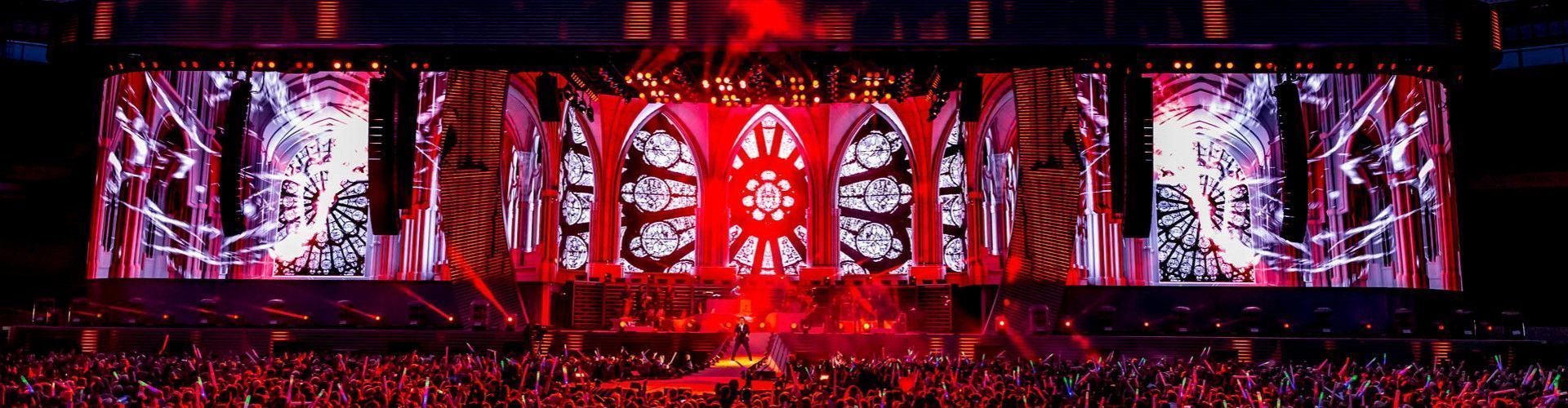This wide-angle, panoramic photo captures a vibrant nighttime concert set in an indoor venue, bathed in warm red and pink hues from the stage lights and projectors. A man, slightly obscured by the distance, stands center stage in a black suit, performing amidst a sea of thousands of enthusiastic fans. The backdrop is a visually striking digital depiction of a Catholic church's stained glass, featuring at least seven distinct panels. The central five panels showcase a prominent circular design with smaller circles and sun-like rays, flanked by panels that evoke floral petal patterns. The atmosphere is electric, with fans waving hands and glow sticks of purple, red, and green, while a light smoky haze adds to the mood. The intricate lighting and detailed stained-glass visuals enhance the overall immersive experience of the concert.